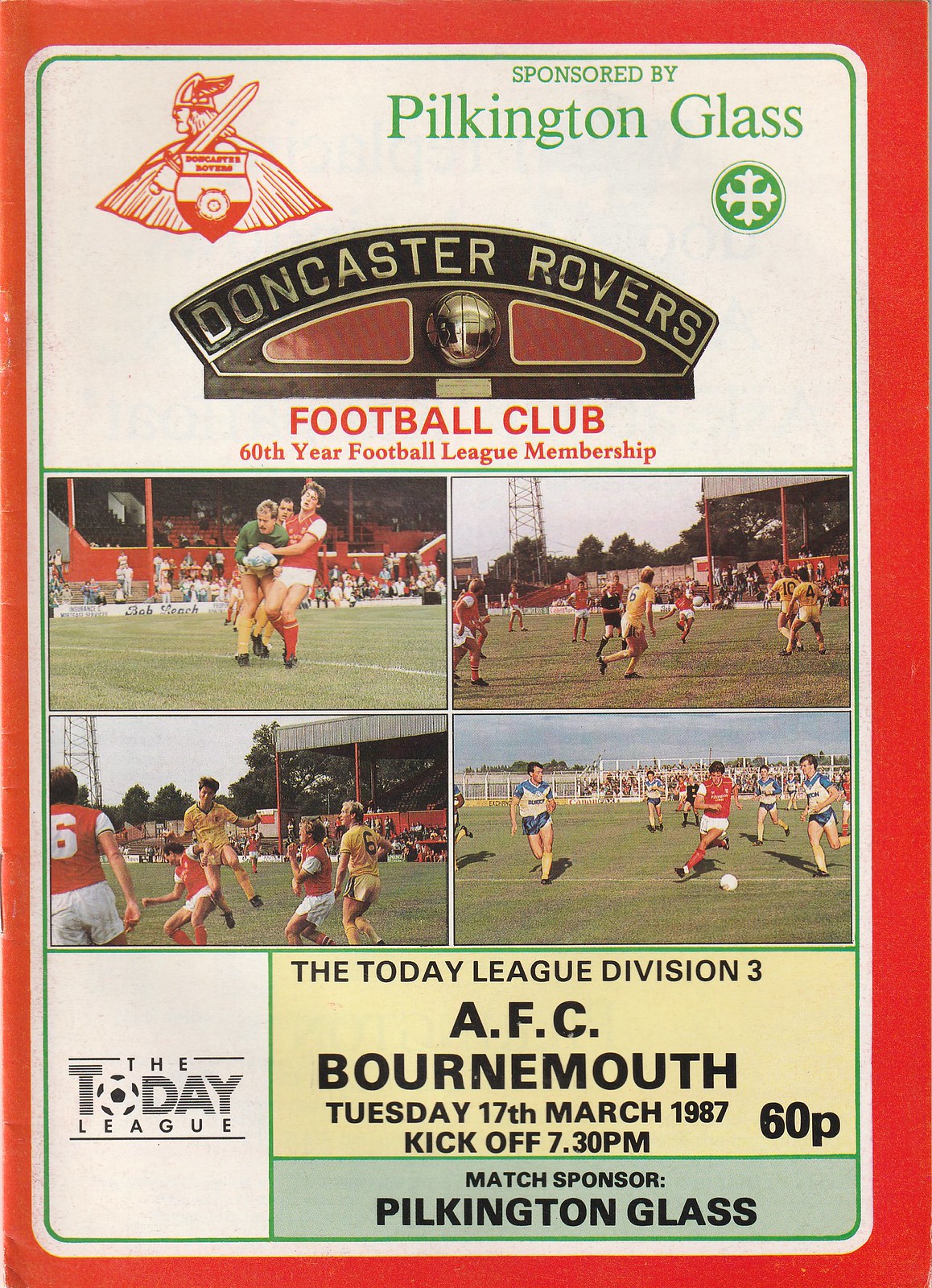The image appears to be an advertisement or program cover for a soccer match, specifically for the Doncaster Rovers Football Club, which is celebrating its 60th year of Football League membership. The advertisement is framed in red and prominently features the sponsorship by Pilkington Glass. At the top, it reads "Sponsored by Pilkington Glass" followed by "Doncaster Rovers Football Club, 60th Year Football League Membership."

The layout includes four quadrants containing vintage photographs of players in action on the soccer field, clad in red shirts with white shorts and short sleeves. Behind them, a red fence can be observed, marking off sections with more of the stadium and spectators visible in the background.

In the lower portion of the image, the left side features the logo for "The Today League," with the O in "Today" depicted as a soccer ball. The right side specifies details of the upcoming match: "The Today League Division III, AFC Bournemouth, Tuesday, 17th March 1987," with kickoff scheduled for 7:30 p.m. The ticket price of 60p is also indicated, along with a note at the bottom right mentioning "Match Sponsor Pilkington Glass."